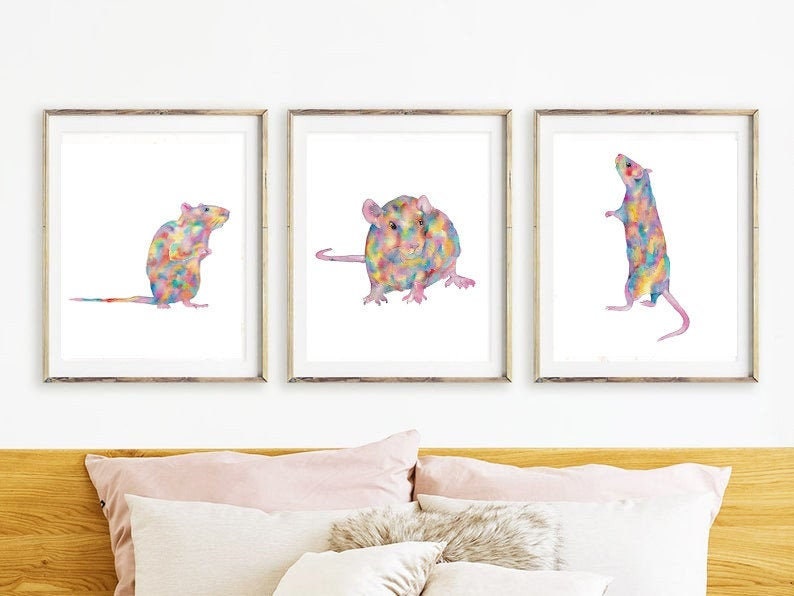The photograph features a neatly arranged bedroom centered around a wooden headboard with various pillows. There are two pink European pillows at the back, followed by two white standard pillows. In front of them is a brownish fur pillow with white tips. Completing the ensemble are two smaller decorative pillows in the front. Above the wooden headboard on the white wall are three equal-sized, gold-framed pictures of a multicolored mouse in different poses. The leftmost image captures the mouse, vibrant with reds, yellows, greens, blues, pinks, and purples, sitting up and looking to the right. The central image shows the mouse on all fours, looking directly at the viewer. The rightmost image features the mouse standing on its hind legs with its tail outstretched, gazing to the left.